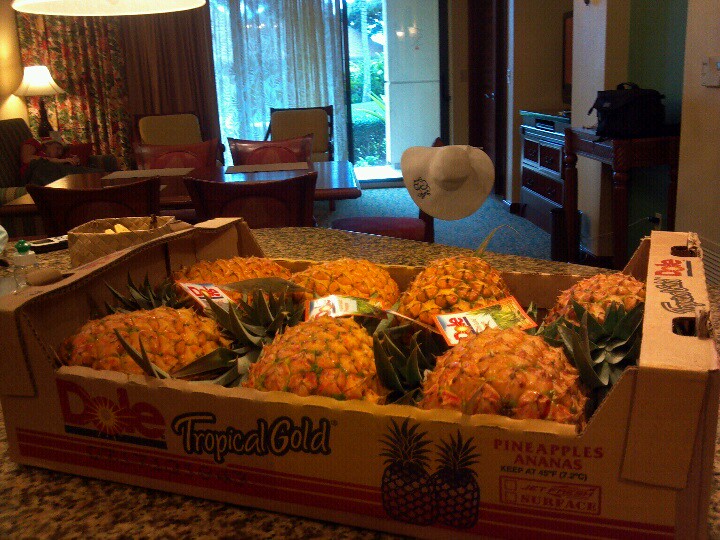This indoor photograph depicts a kitchen setting with a box of seven ripe, golden-yellow pineapples placed on a large granite countertop island. The cardboard box is an open crate with sides and features the Dole brand logo with red letters, a sun rising from the letter 'O,' and an underline. It also reads "Tropical Gold" and "Pineapples Ananas," accompanied by images of pineapples and a stamp indicating "jet surface." The image, captured in low lighting, shows a table set up in the background, likely in a living room, surrounded by red leather chairs. Additionally, a nearby wooden dining table with five chairs, a lit lamp in the corner, flowery curtains, and a glass screen door peering into a green garden courtyard add to the scene's cozy ambiance.